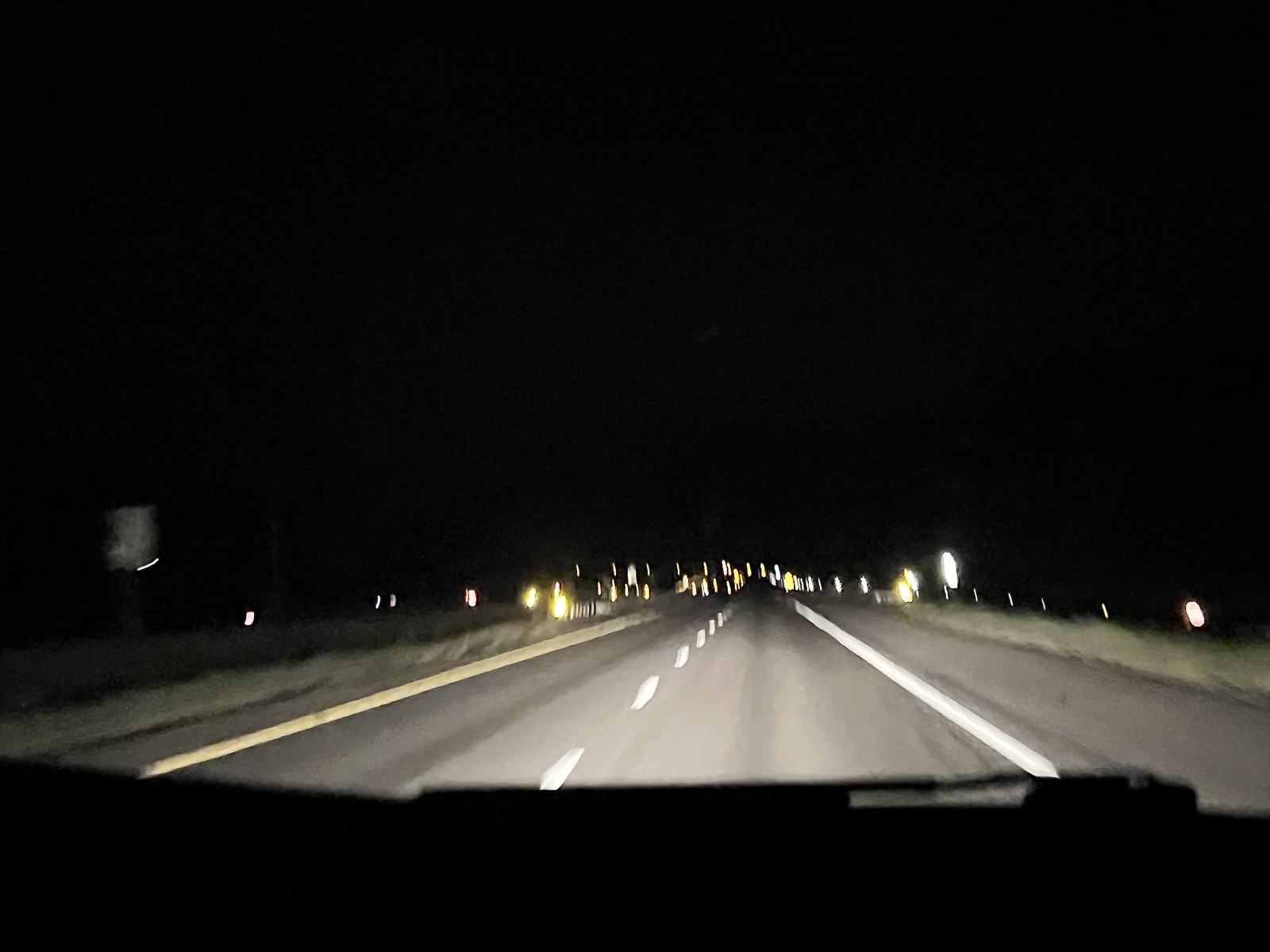This nighttime photograph, taken from inside a moving vehicle, captures the view through the front windshield. The car's dashboard is partially visible at the bottom, along with the outline of one windshield wiper. The vehicle is traveling down a two-lane highway on the right-hand side of the road. The scene is illuminated by the car’s headlights, highlighting the center white lines of the road, which appear streaky due to the motion. Reflective surfaces, likely road signs or guardrails, stand out on both sides of the road. A concrete barrier and a narrow strip of grass with lined reflectors run parallel to the highway, while a potential building or road sign is faintly visible on the right. The sky is pitch black without visible stars or moon, adding to the overall darkness of the scene. There are no other vehicles on the road, emphasizing the solitude and motion in this nighttime journey.